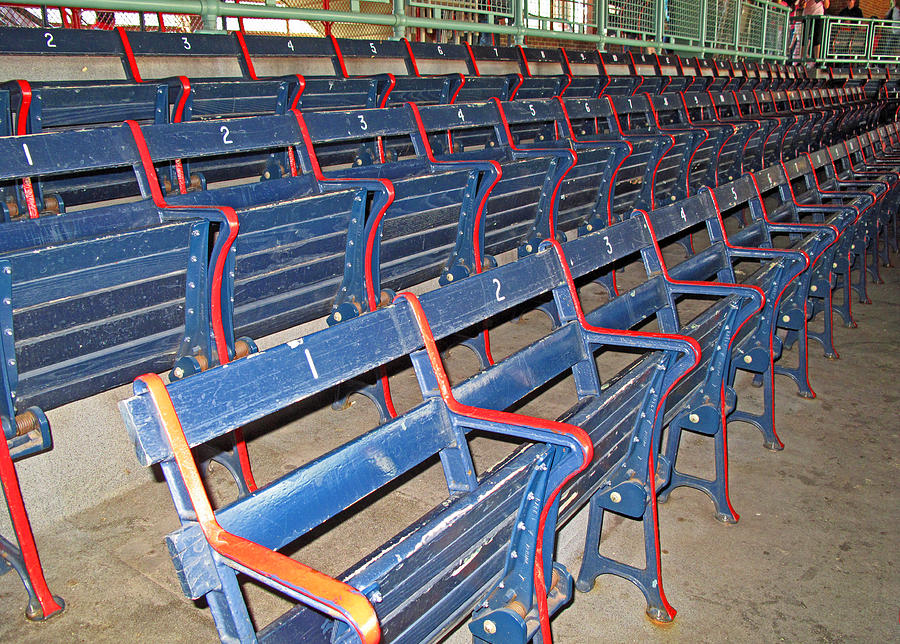This image captures the arranged interior of a stadium, focusing on its aging yet vivid seating. The blue wooden benches, noticeably worn and chipped from extensive use, form three parallel rows, each marked with ascending numbers starting at one for clarity. Red-painted arms or dividers separate the individual seats, although much of this paint has worn away, exposing the bare wood beneath. Below the benches, the grounding is a rather grimy concrete, adding to the overall atmosphere of weathered utility. The tiered seating is visually framed by a bright green fence, serving as a barrier at the top of the image. This fencing suggests a designated area for standing spectators, allowing them to enjoy refreshments without missing the ongoing game. In the distant background, higher levels of seating can be seen, populated by a few people, further enhancing the sense of an expansive and well-used venue.